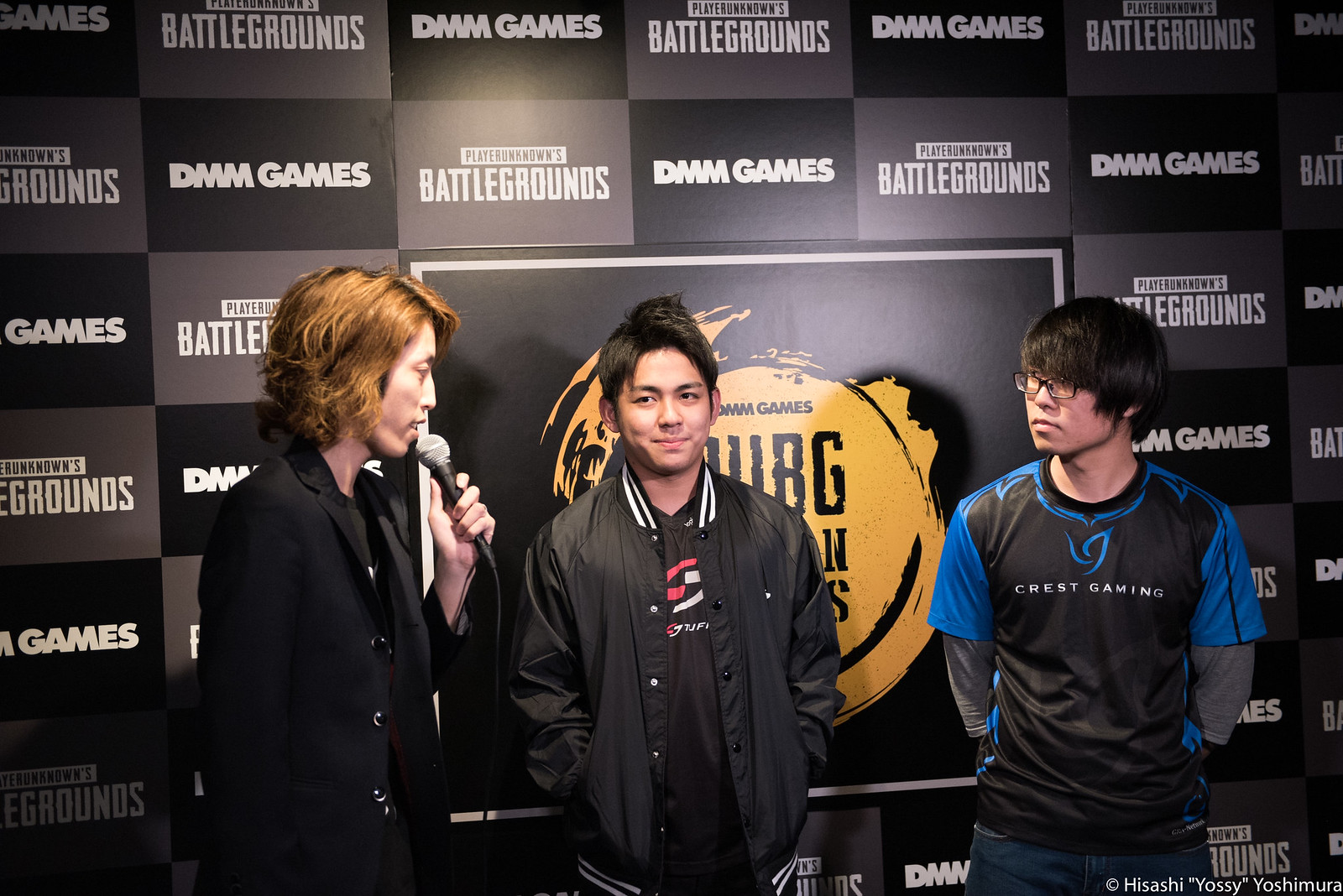In the image, three men are standing in front of a banner at a gaming event, featuring the text "DMM Games PlayerUnknown's Battlegrounds" in white against a black and gray background with accents of yellow. The man on the left, with short red hair, is holding a black and gray microphone and is seen in side profile as he talks to the other two. He's wearing a black suit jacket. The man in the center, facing the camera head-on, sports a black and white jacket over a black, white, and red undershirt. The man on the right has black hair and is also facing the camera. He wears a black and blue shirt over a gray long-sleeve shirt and blue jeans, with "Crest Gaming" printed on his chest. All three have pale peach-colored skin. The entire background is covered by the event banner, emphasizing the professional, interview-like setting, and in the bottom right, there is a copyright notice for Hisashi Yoshimura.